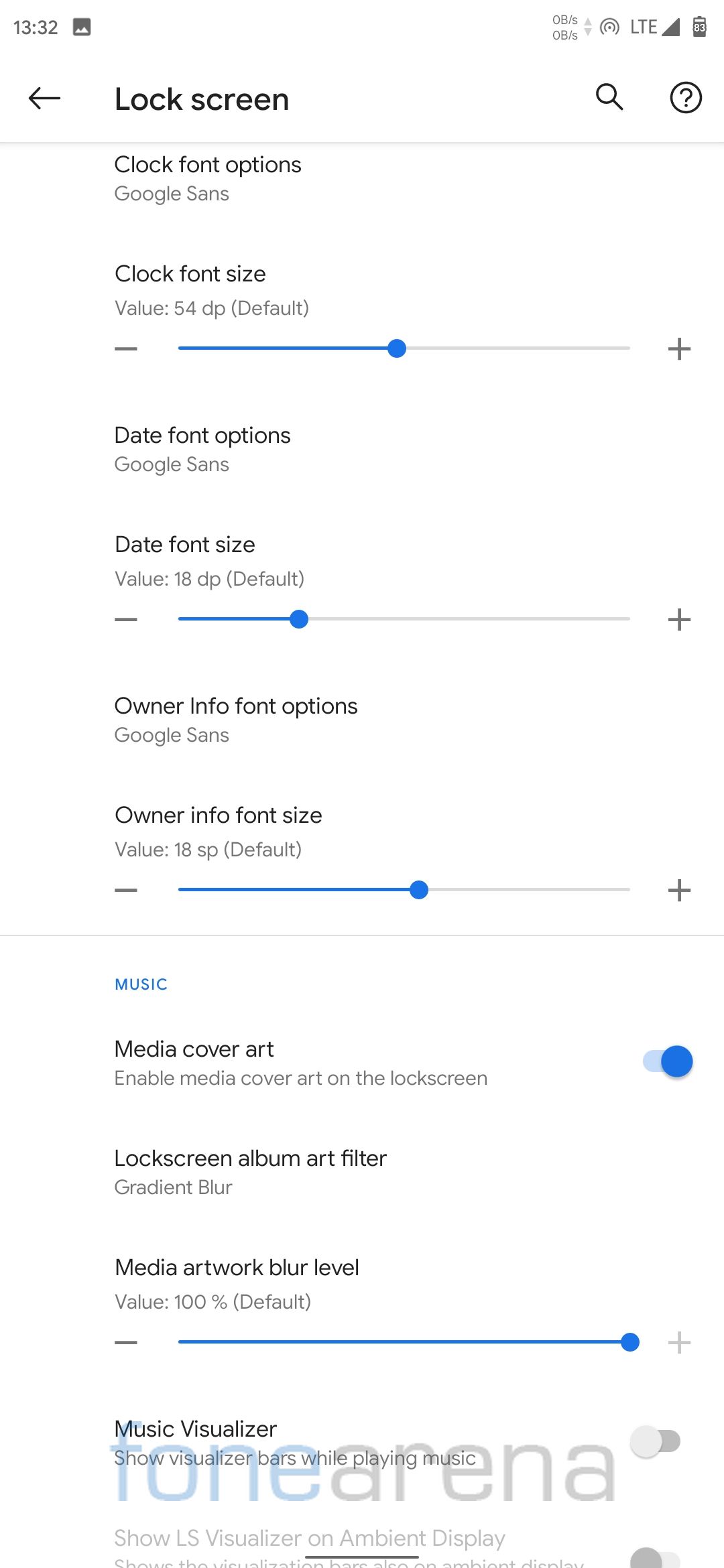This screenshot captures a section of a smartphone's settings menu, specifically focusing on lock screen customization options. At the top, the image is marked with the identifier "121332." The upper right corner shows icons representing LTE signal strength and battery status. The background is predominantly white with black font, indicating a typical interface for phone settings.

Prominently displayed, the menu begins with navigation indicators such as an arrow, a magnifying glass, and a question mark inside a circle. The first setting listed is "Lock Screen Clock Font Options," featuring the "Google Sans" font and a default clock font size of "54 DP." Following this, the "Date Font Options" also uses the "Google Sans" font with a default size of "18 DP."

Additional settings include "Owner Info Font Options," again using "Google Sans" with a default size of "18 SRDP." Under the "Include Music and Media Cover Art" section, there is an option to enable media cover art on the lock screen, accompanied by a blue toggle switch indicating it is active. The "Lock Screen Album Art Filter" is set to "Gradient Blur," with the blur level set at "100%," demonstrated by a blue bar and circle slider along with a gray plus sign.

Further options involve the "Music Visualizer" to show visualizer bars while playing music, paired with a gray circle indicating it is disabled. Another option is "Show L Visual on Ambient Display," also indicated by an inactive gray circle.

At the bottom of the screenshot, a watermark is present, consisting of colors white, black, blue, and gray, with the text "Phone Arena" stylized as "F-O-N-E arena."